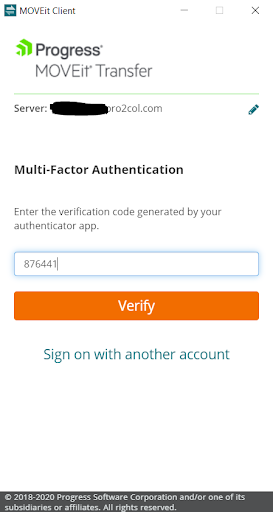The image is a screenshot of an authentication page for a service called MOVE IT CLIENT. In the upper left portion of the image, there is a square icon with a dark teal background featuring a pair of half arrows in the center. Next to the icon, the company's name, "MOVE IT CLIENT," is displayed in black text, with "MOVE" in all capital letters. The background of the page is white.

Below the MOVE IT CLIENT header, there is another icon on the left side showing three progressively smaller, green carrot-shaped arrows. Next to this icon is the word "PROGRESS," followed by "MOVE IT TRANSFER" directly below it.

There is a section labeled "Server" with some information blacked out, likely to conceal personal data. A part of an email address is visible next to the blacked-out section, suggesting the redacted area contains a username or personal identifier.

Further down, the text "MULTIFACTOR AUTHENTICATION" is prominently displayed in bold black font. Below this, a dark gray instruction reads "ENTER THE VERIFICATION CODE GENERATED BY YOUR AUTHENTICATOR APP." There is a text bar under the instruction containing the code "876441."

At the bottom of the section, there is a large, rectangular, orange VERIFY button with white text. Beneath this, a clickable link in blue text reads "SIGN ON WITH ANOTHER ACCOUNT."